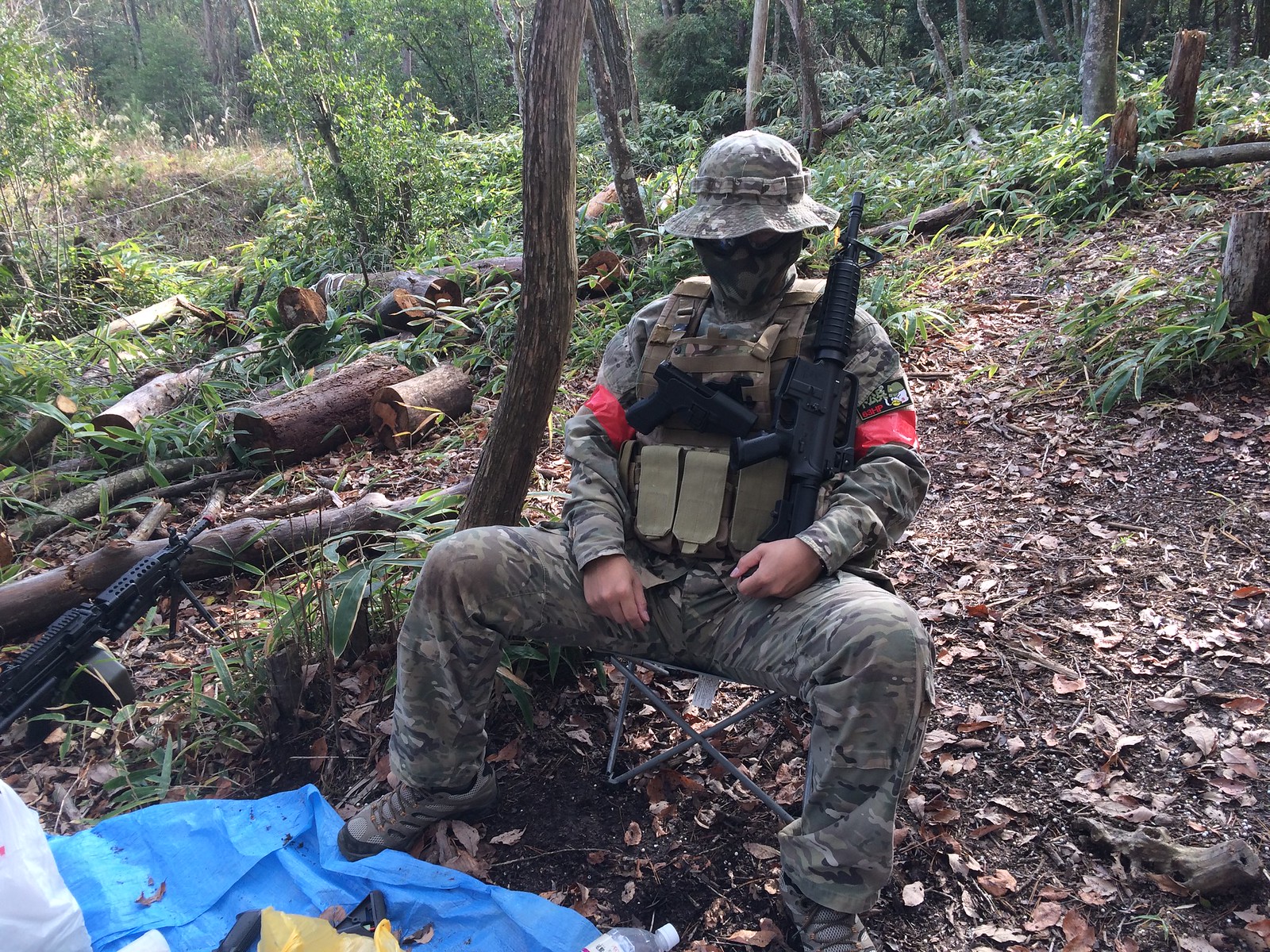In the midst of a dense forest, with fallen logs and a carpet of leaves and grass, a man sits cross-legged on a chair, fully attired in a green camouflage uniform. His outfit includes a matching camouflage top, pants, hat, and a mask that conceals his face, leaving only his eyes visible. Across his chest lies a vest equipped with compartments, housing a short pistol. He holds a long black gun in his left hand, resting it against his body. A canteen hangs on his side, and a blue tarp lies by his feet. The background showcases numerous trees, standing tall and casting shadows, with the ground littered with dead leaves and scattered wood logs.